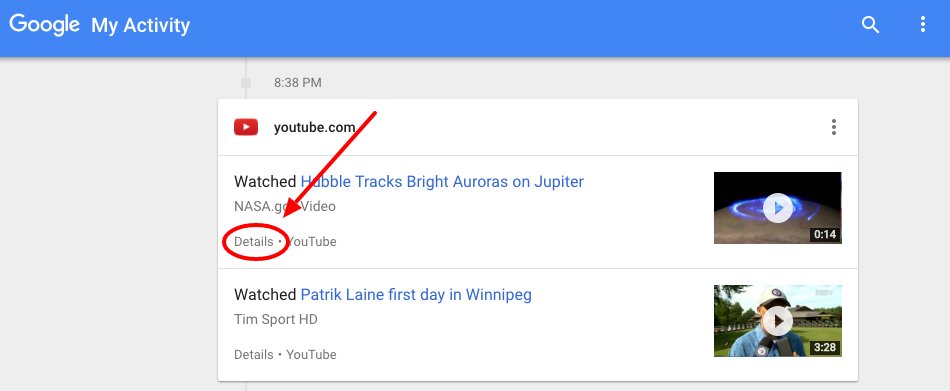This image is a detailed screenshot of someone's Google My Activity page. 

At the top of the image, there is a blue title bar with the text "Google" prominently displayed in white with a capital "G," followed by "My Activity" also in white with capital "M" and "A." On the far right of this title bar, there are two icons: a magnifying glass for search and a vertical ellipsis (three dots) for more options.

Beneath the title bar is a gray rectangular box displaying the time "8:38 p.m." Directly below this is a smaller white rectangular box featuring the YouTube logo, a red play button, and the text "YouTube.com," followed by another vertical ellipsis for more options. 

Within this white rectangular box, there is a horizontal gray line separating different sections. The text "Watched: Hubble Tracks Bright Auras on Jupiter - NASA Video" is prominently displayed. Surrounding this text is a red circle with a red arrow pointing towards it from the upper right (one o'clock position), indicating its significance. To the right, an image of a thumbprint and a play button icon are visible.

Following this section, there is another entry indicating a watched video titled "Patrick Lane - First Day in Winnipeg," uploaded by the channel TimSportHD. This is denoted with "details.YouTube" and is accompanied by another thumbprint image, a play button, and the video's timestamp.

This image carefully showcases the user's recent YouTube activity with structured, time-stamped entries depicted in a clean and organized interface.